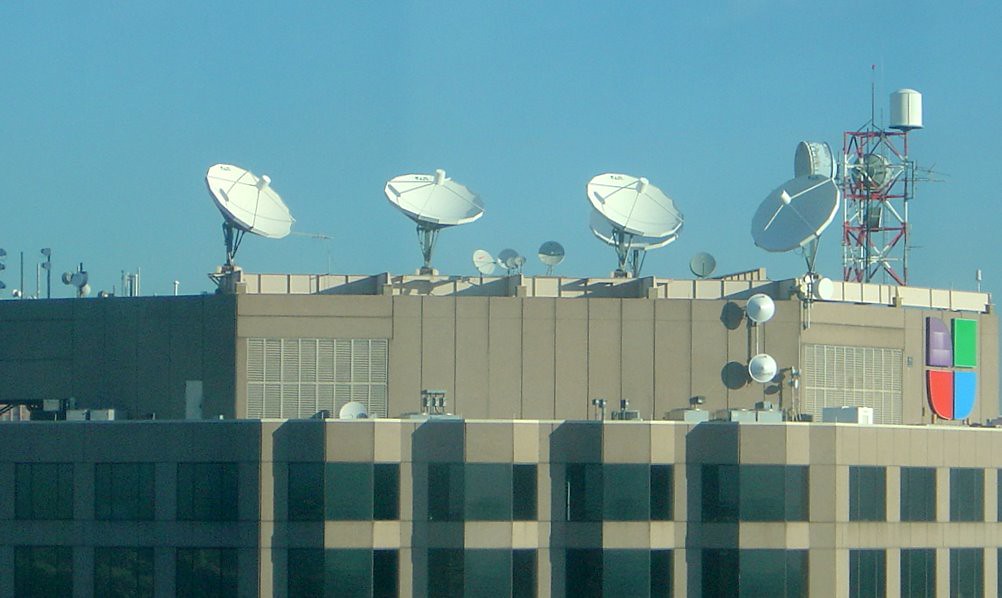This image depicts the rooftop of a tall building, identifiable as the Univision headquarters due to its distinctive logo featuring purple, green, red, and blue colors. The rooftop is densely populated with a variety of communication equipment, including very large parabolic dishes, satellite antennas, microwave antennas, and smaller satellite dishes of various sizes, indicating it is a hub for broadcasting and communication. The building has a medium brown, almost slate gray exterior with dark, tinted windows. There is a notable additional tower on the rooftop equipped with omnidirectional antennas and further parabolic dishes, suggesting ground-based transmission capabilities. The sky is clear with a subtle haze, underlining a sunny day. The overall setup points to the building's role as a significant communication center, possibly for media transmission or scientific research.